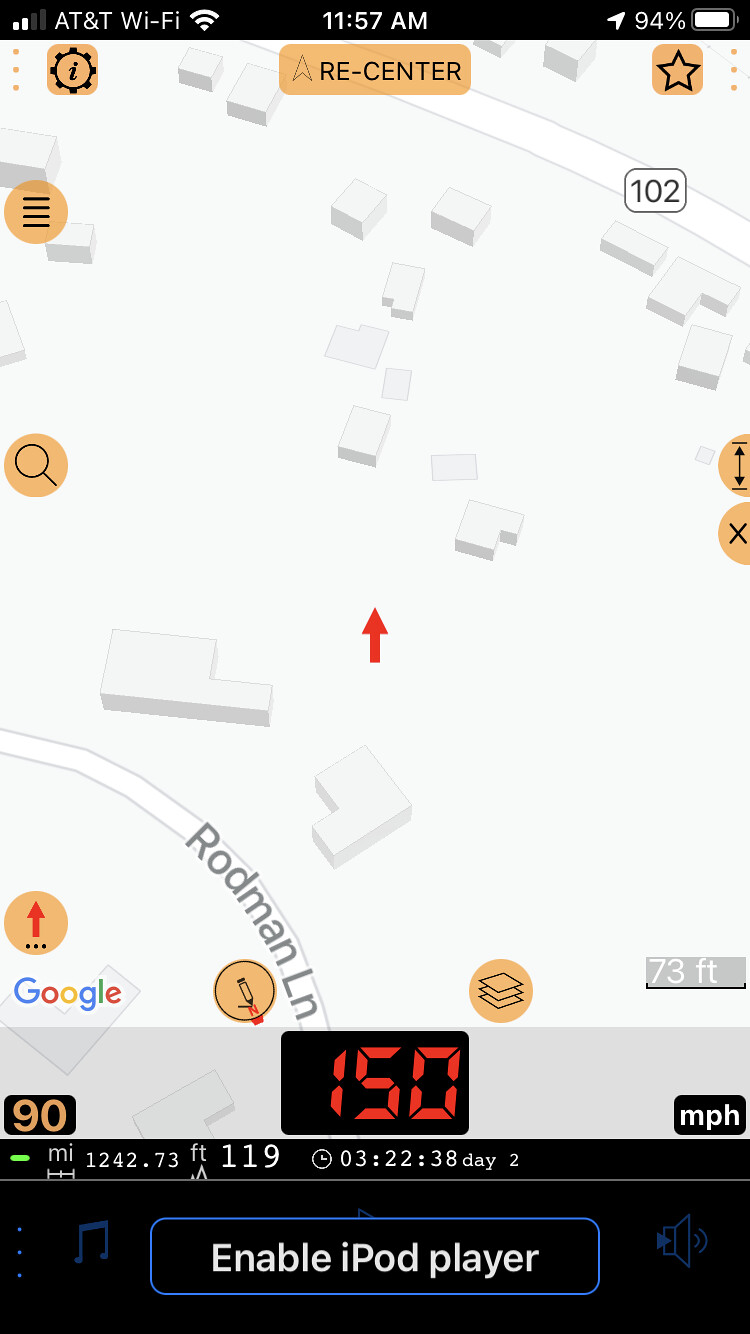The screenshot showcases a phone screen displaying a map application, complemented by a music player interface at the bottom. The rectangular image has longer sides on the left and right compared to the top and bottom edges. 

At the very top of the screenshot, a black banner runs along the edge, containing multiple lines of black text and symbols. Starting from the left, the banner features a signal strength indicator with four bars, ranging in height from shortest to longest — two bars are white, and two are gray. Next to this, in all capital letters, reads "AT&T," followed by "Wi-Fi" and an icon resembling an upside-down triangle composed of curved lines. Centered on the banner is the time "11:57 AM," and on the right side, a horizontal, fully white battery icon displays "94%."

In the center top area of the map, an orange rectangle labeled "Re-center" stands out. The top left corner of the map features a cogwheel icon accompanied by a cursive lowercase "i," while the top right corner displays a five-pointed black star outline. The map itself has a predominantly gray color scheme.